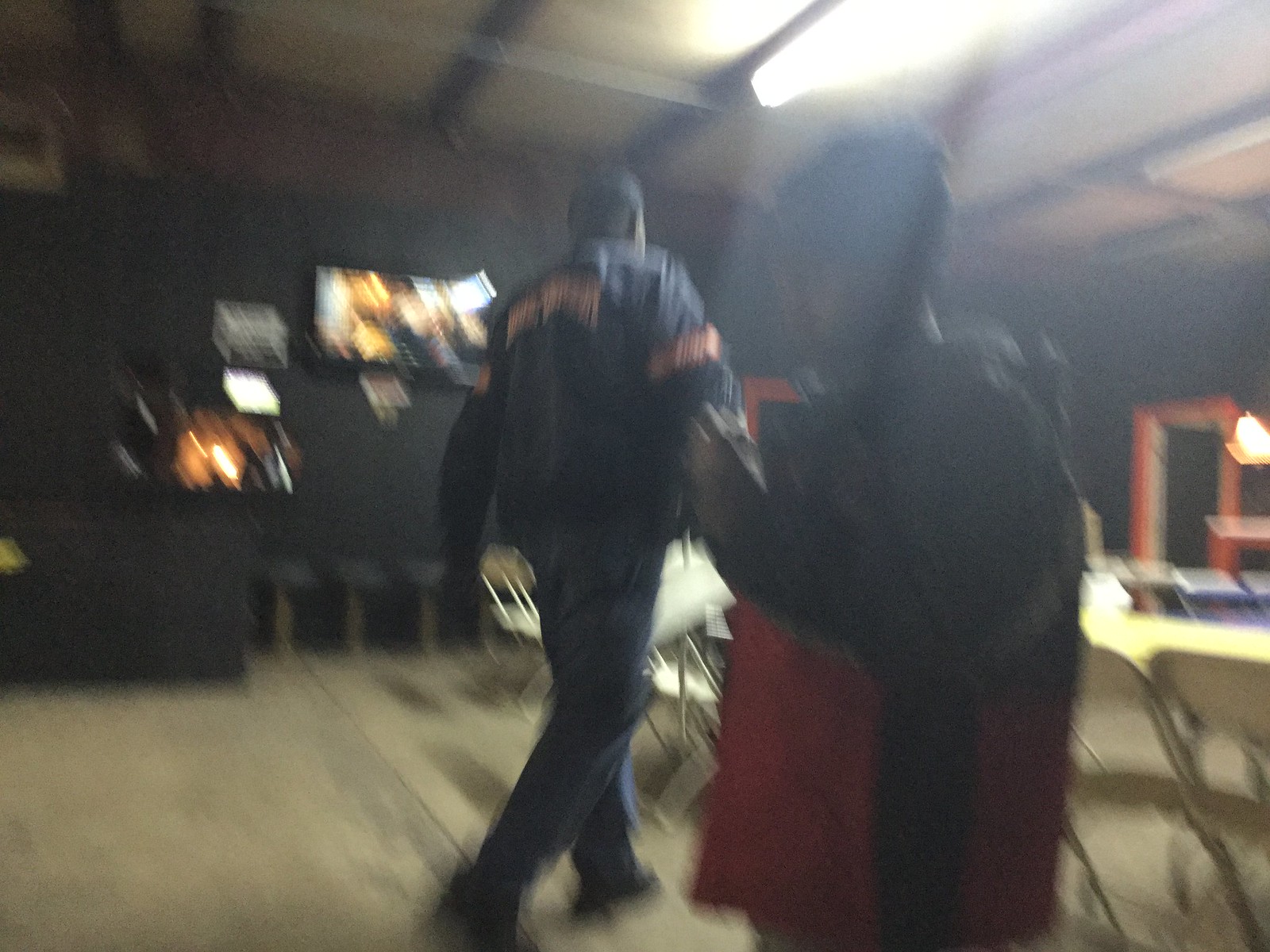In a blurred photograph of a meeting room, two black men are captured in what appears to be a gathering or discussion. The back wall of the room is black and adorned with indiscernible screens or photographs. To the right, a white table set with folding chairs—some clearly visible while others are partially obscured—provides a structured backdrop. The ceiling, painted gray, hosts a barely visible fluorescent light fixture. 

In the middle of the image, one man, dressed in a black jacket featuring a white and red print, jeans, and black shoes, faces away from the camera. Closer to the front, the second man stands out in a stylish red and black jacket, paired with a gray or black hat and possibly glasses. He appears focused on his phone, indicating an informal setting amidst the room’s formal arrangement.